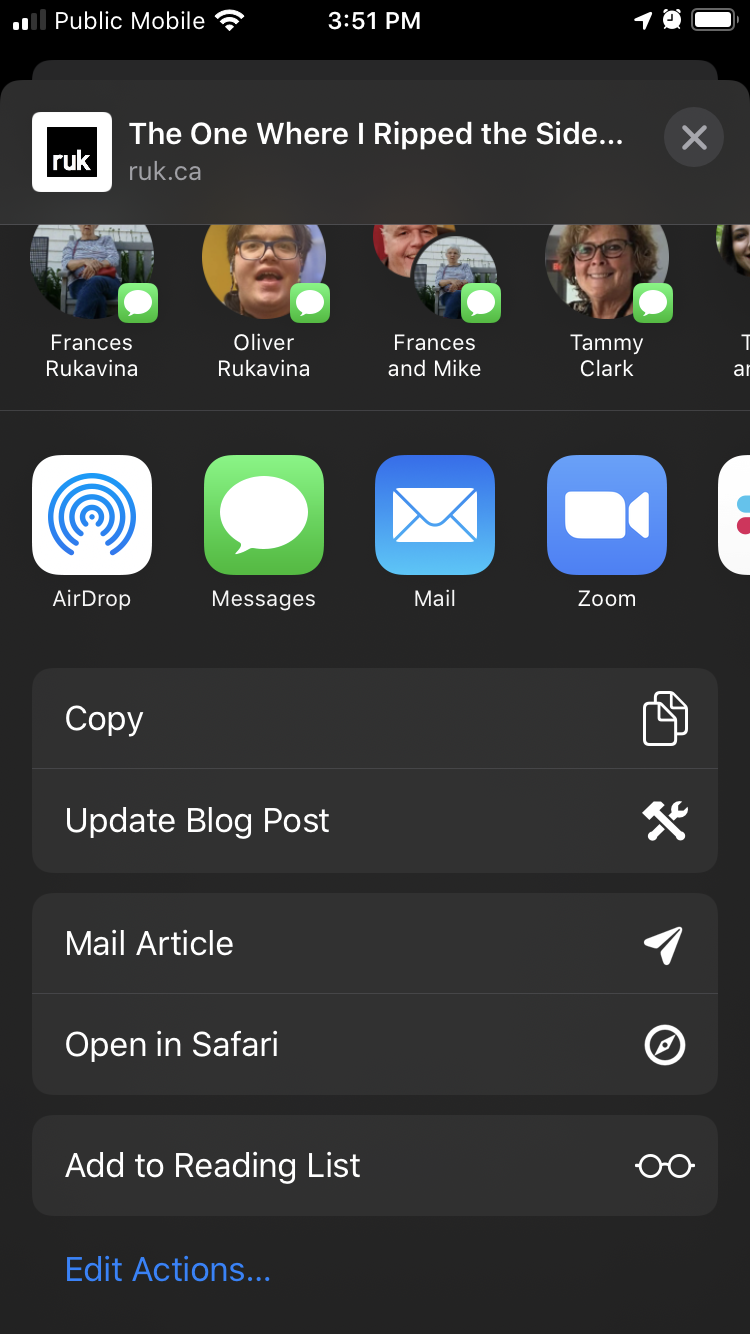The image depicts a screenshot from an iPhone displaying the sharing options in the Safari browser. At the top, there's a partially visible URL "ruk.ca," indicating a Canadian top-level domain. The interface is set to a dark theme, with a black background. Below the URL, there are multiple sharing options and a list of recent messaging contacts, including Francis, Oliver, Francis again, and Tammy.

The screen features a series of icons corresponding to various actions. For instance, the 'Copy' option is represented by an icon of two overlapping pieces of paper. Other available actions include Airdrop, Messages, Mail, Update Blog Post, Mail Article, Open in Safari, and Add to Reading List. This suggests that the user is either sharing the article or exploring the additional options available for interaction with the content in Safari.